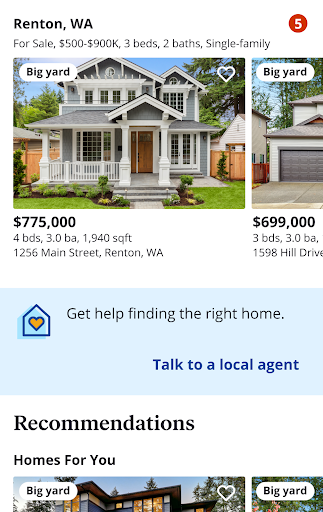This image displays several property listings for houses in Renton, Washington. In the upper left corner, there is a listing for a single-family home priced between $500,000 and $900,000, featuring three bedrooms and two bathrooms. A notable feature highlighted is a "big yard," denoted by a red circle with the number five in white. Adjacent to this is a photograph showcasing the expansive yard, while another photo, less visible, indicates a property priced at $775,000. This house offers four bedrooms, three bathrooms, and spans 1,940 square feet, located at address 1256 Maine, Renton, Washington.

Another listing mentions a "big yard" and is priced at $699,000, featuring three bedrooms and three bathrooms, located at 1598 Hill Drive. Below these listings, there is a section encouraging users to "Get help finding the right home." The phrase "Talk to a local agent" is highlighted in blue on a light blue background with a red heart inside a house symbol. 

Further down, the section labeled "Recommendations" and "Home for you" contains two partially cut-off photos, both emphasizing "big yard" in the upper left corner. The prominent colors throughout the images are brown, green, red, white, black, gray, and blue.